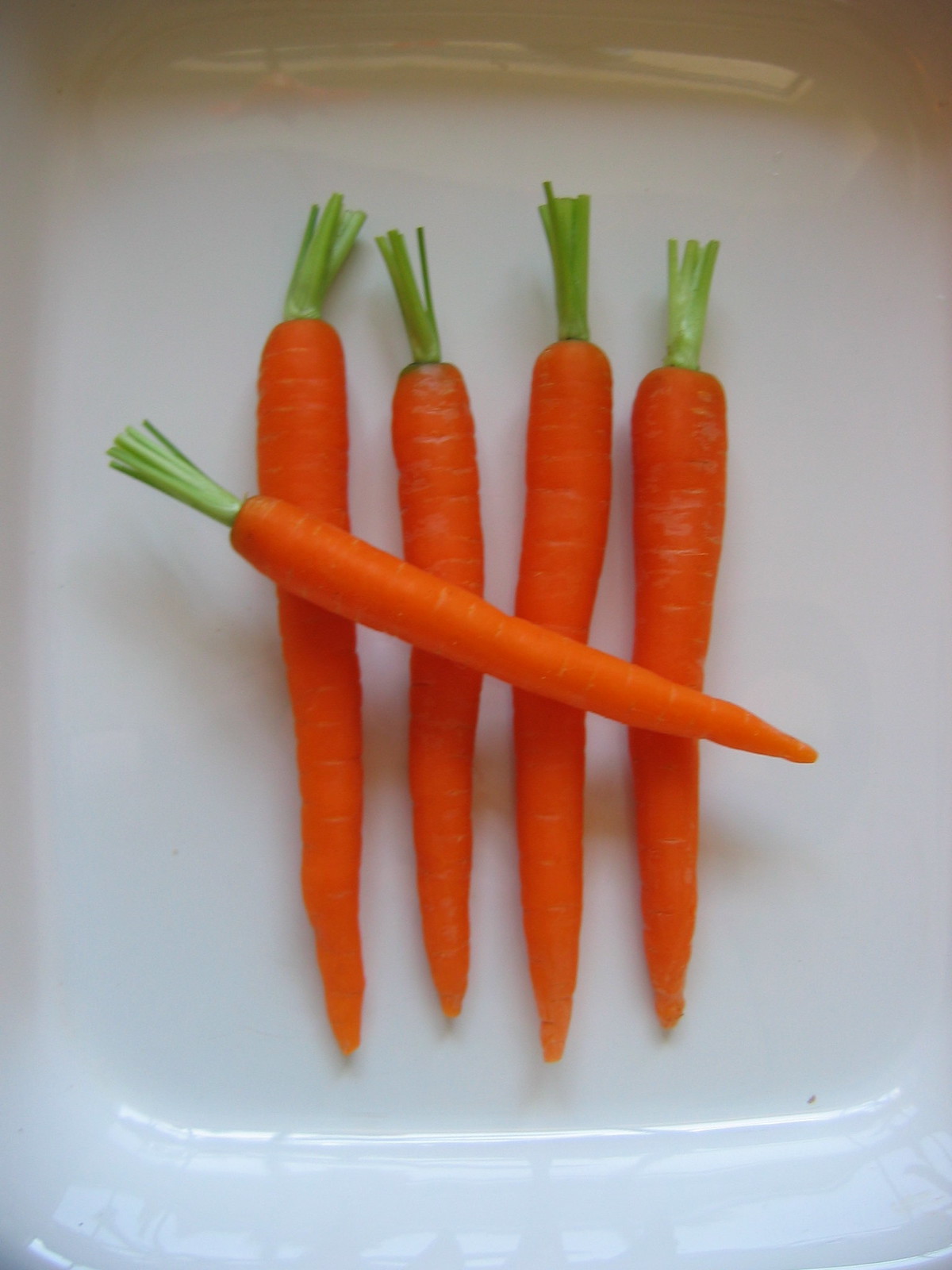A photograph shows a white, rectangular casserole dish containing five bright orange carrots. Four of these carrots are laid out vertically, with their pointy ends facing downward and their green stalks, which are neatly trimmed, positioned at the top. Diagonally across these four carrots lies a longer, skinnier carrot, creating a crisscross pattern reminiscent of a tally mark. The dish, captured from a close distance, reveals a slight glare from an overhead light source reflecting on its white surface, with shadows cast by the diagonal carrot adding depth to the composition. The carrots appear pristine and clean, with their vivid orange color contrasting sharply against the white casserole dish.